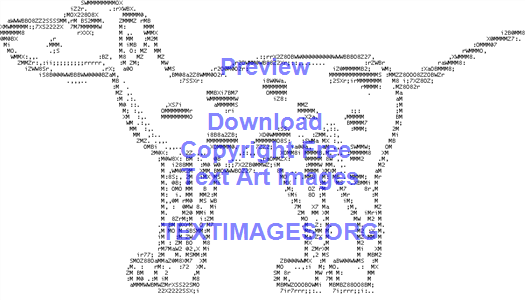The image features a minimalistic, digitally produced ASCII-style representation of a dog, created using characters from a typewriter or keyboard. The dog is facing left, with its head forward to the left and its tail pointing up and to the right. The depiction is in black font, with the intricate arrangement of letters forming the dog's outline, complete with visible details such as one eye, a nose, ears, four legs, and black spots. Superimposed over the center of the dog is a watermark in blue font reading "preview," followed by the phrases "download copyright free text art images" and "textimages.org" in capital letters. The entire composition is set against a solid white background, suggesting it to be a stock or clipart image. The scene emphasizes the central placement of the ASCII dog and the watermark text with no other objects in view.